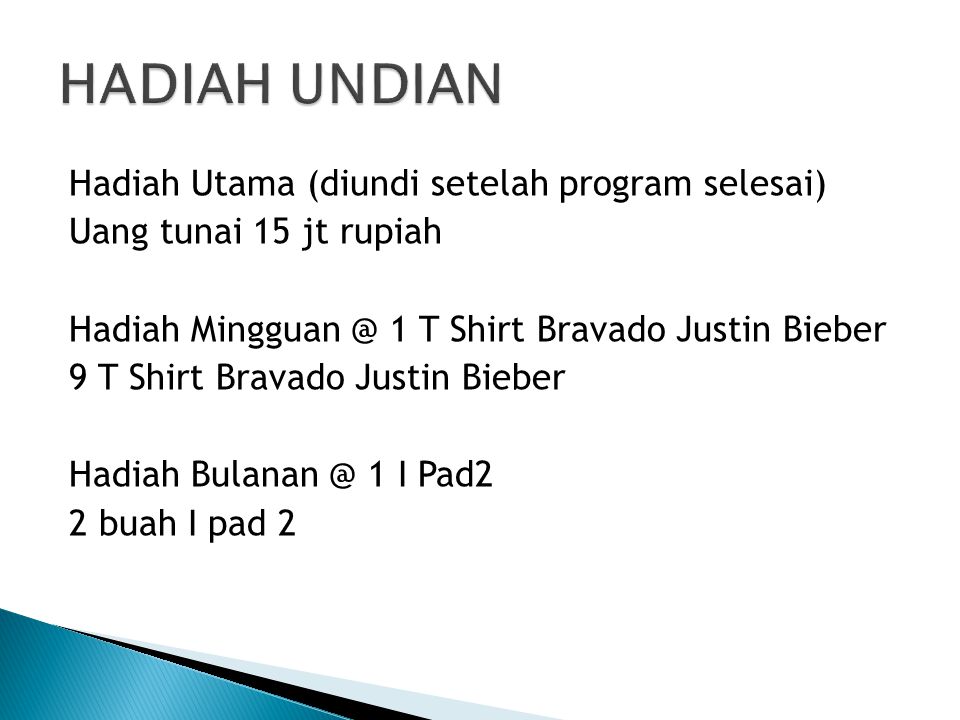The image features a primarily white background with mostly text in a language that is not English, potentially Indonesian. The largest text at the top reads "HADIA UNDIAN," and below it, in smaller fonts, are several sections of text. The first section reads "HADIA UTAMA," with a parenthetical note saying "DIYUNDI SAAT PROGRAM SELESAI," followed by "UANG TUNAI 15 JT RUPIAH," which suggests a main prize of cash worth 15 million Rupiah. Another section mentions "HADIA MINGGUAN" featuring "1 T-SHIRT BRAVADO JUSTIN BIEBER" and "9 T-SHIRT BRAVADO JUSTIN BIEBER," indicating weekly prizes of Justin Bieber t-shirts. The final section lists "HADIA BULANAN" with "1 iPad 2" and "2 BUA iPad 2," suggesting monthly prizes of iPads. In the lower left-hand corner, there are three expanding triangles: a blue one in the front, a black one in the middle, and a light blue one in the background. The overall composition suggests it is an advertisement for a giveaway or promotional event involving cash, branded t-shirts, and iPads.